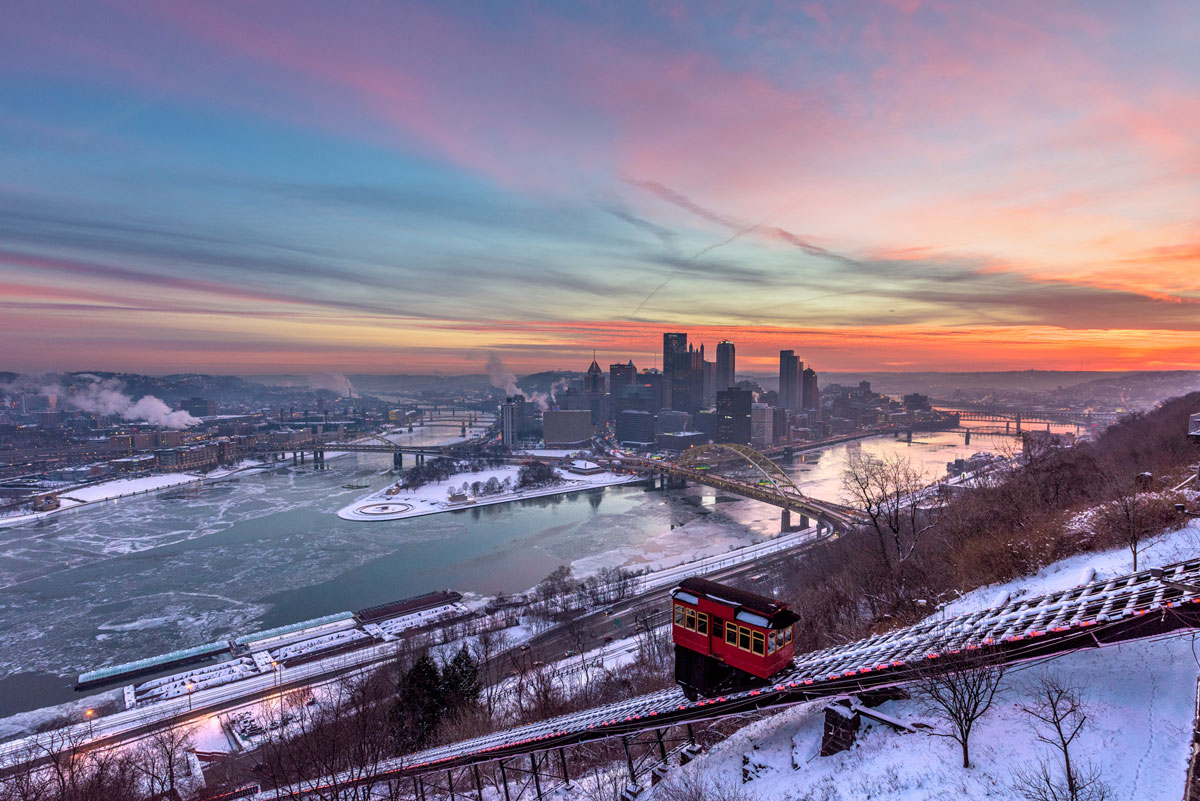The image depicts a cold cityscape under a picturesque sky streaked with pink, blue, orange, and yellow hues from the setting or rising sun. A steeply sloped track runs diagonally, featuring a red and black trolley with a black top, six arched windows with yellow frames, and a central door. Supported by a triangular black surface, the trolley remains level as it ascends or descends the railway. Below, a river with light green water and white foam flows around a cluster of gray skyscrapers in the heart of the city. The scene includes several bridges spanning the waterway, including one brown bridge prominent in the middle distance. On the far left, an industrial area emits white and light gray smoke, which drifts to the left. Trees dusted with white snow dot the landscape, enhancing the wintry atmosphere.